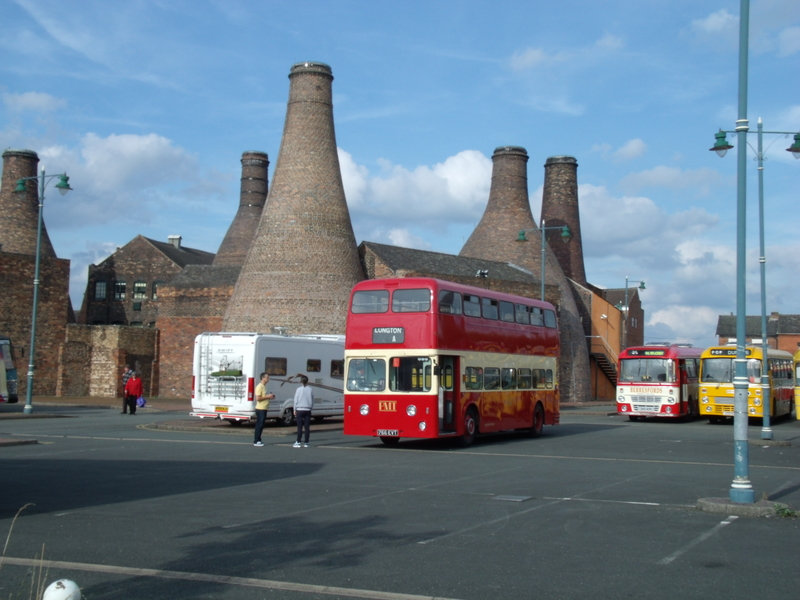This color snapshot photograph, likely from an old film camera, captures a bright sunny day in a cityscape defined by historical architecture and bustling activity. The background is dominated by intricate, antiquated brick buildings adorned with unique, wine bottle-shaped chimneys that resemble smokestacks. Among the light shadows creeping into the frame, a vast blacktop parking lot stretches out, dotted with familiar urban elements. Prominently featured in the center of the image is a glossy red double-decker bus brandishing a white stripe across its middle and lined with windows on its upper deck. Close by, to the left of the bus, a white tour van is parked. The right side of the image reveals two more buses—one red and the other a mustard-yellow hue—parked behind tall, light blue lamp posts that stand sentinel along the horizon, their lamps dangling from horizontal stringers. Additionally, a soccer ball casually rests on the pavement on the left, adding a touch of playfulness to the scene. Amid this urban ensemble, a few pedestrians, estimated to be three or four in number, stand within the wide expanse of the road, contributing to the lively atmosphere of this somewhat out-of-focus yet evocative photograph.